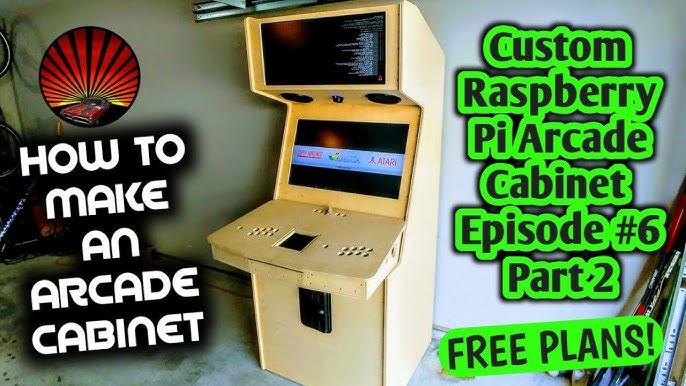The image appears to be a detailed advertisement for building a custom Raspberry Pi arcade cabinet, part of an informational series titled "How to Make an Arcade Cabinet." The scene is set in a white-walled room and features a vintage, upright arcade machine, reminiscent of 1970s designs, with a plain, wooden, light yellow-brown cabinet that looks handmade. A standout element is a logo in the top left corner, depicting a hot rod car driving out of a sunset with yellow, gold, and red stripes. Text overlaying the image includes a white, shadowed title on the left stating, "How to Make an Arcade Cabinet," and green text with black letters on the right that reads, "Custom Raspberry Pi Arcade Cabinet, Episode No. 6, Part 2, Free Plans!" This promotional header is visually engaging, capturing the nostalgic essence of vintage arcade gaming while highlighting the offer of free plans.